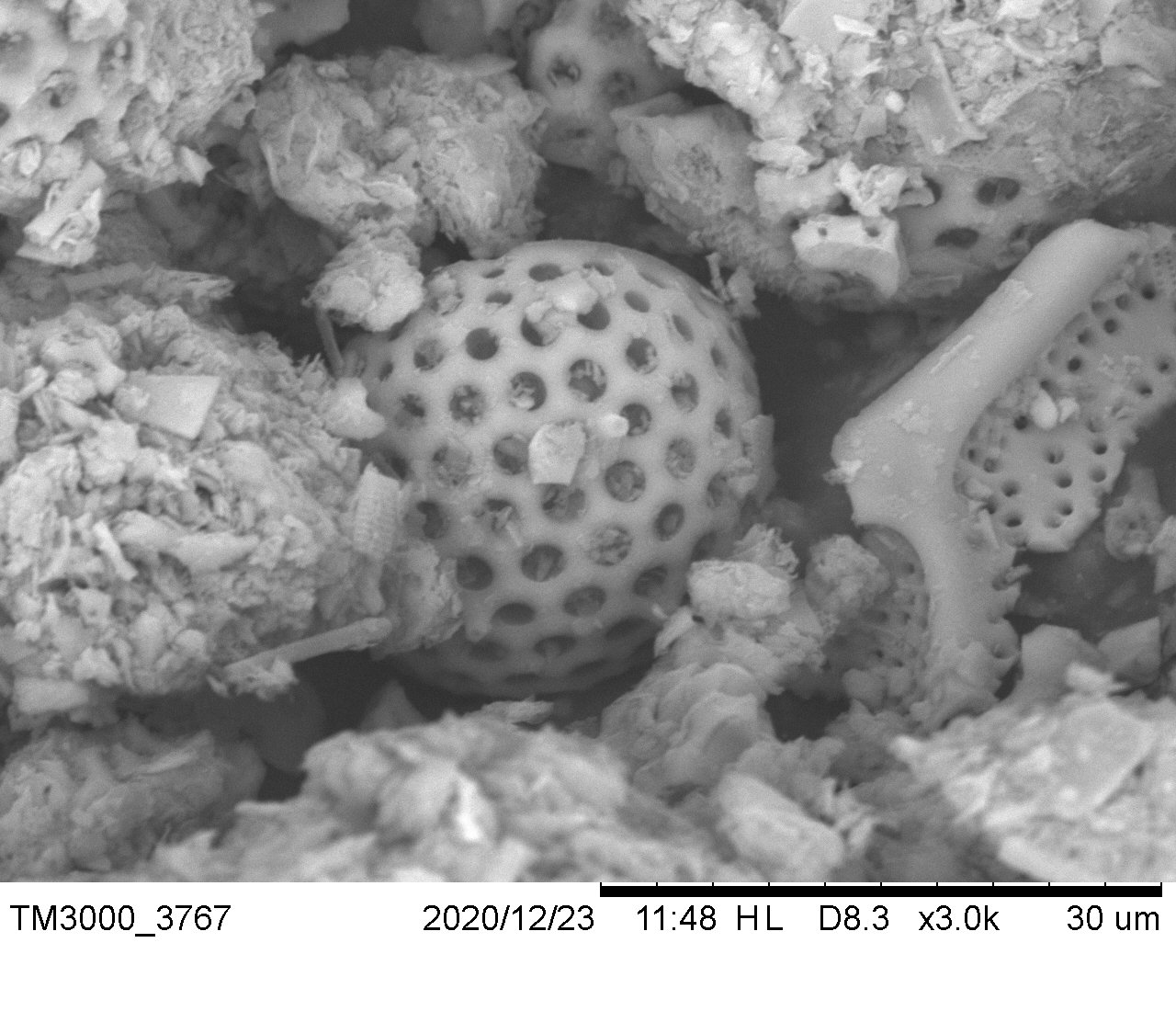The image is a highly detailed black and white photograph, likely taken through a microscope, possibly of parasites, dust mites, cells, or spores. The image, captured on December 23, 2020, zooms in to a magnification level of 3.0K, displaying intricate spongy-like and circular structures with various holes. The particles are shown very close up at 30 micrometers. The bottom left of the image includes the text "TM3000-3767-2020-12-23 1148HL-D8.3-X3.0K-30UM," providing technical details and context. Despite the uncertainty regarding the specific nature of the subject, the image is clear and well-lit, exhibiting a high-contrast grayscale.